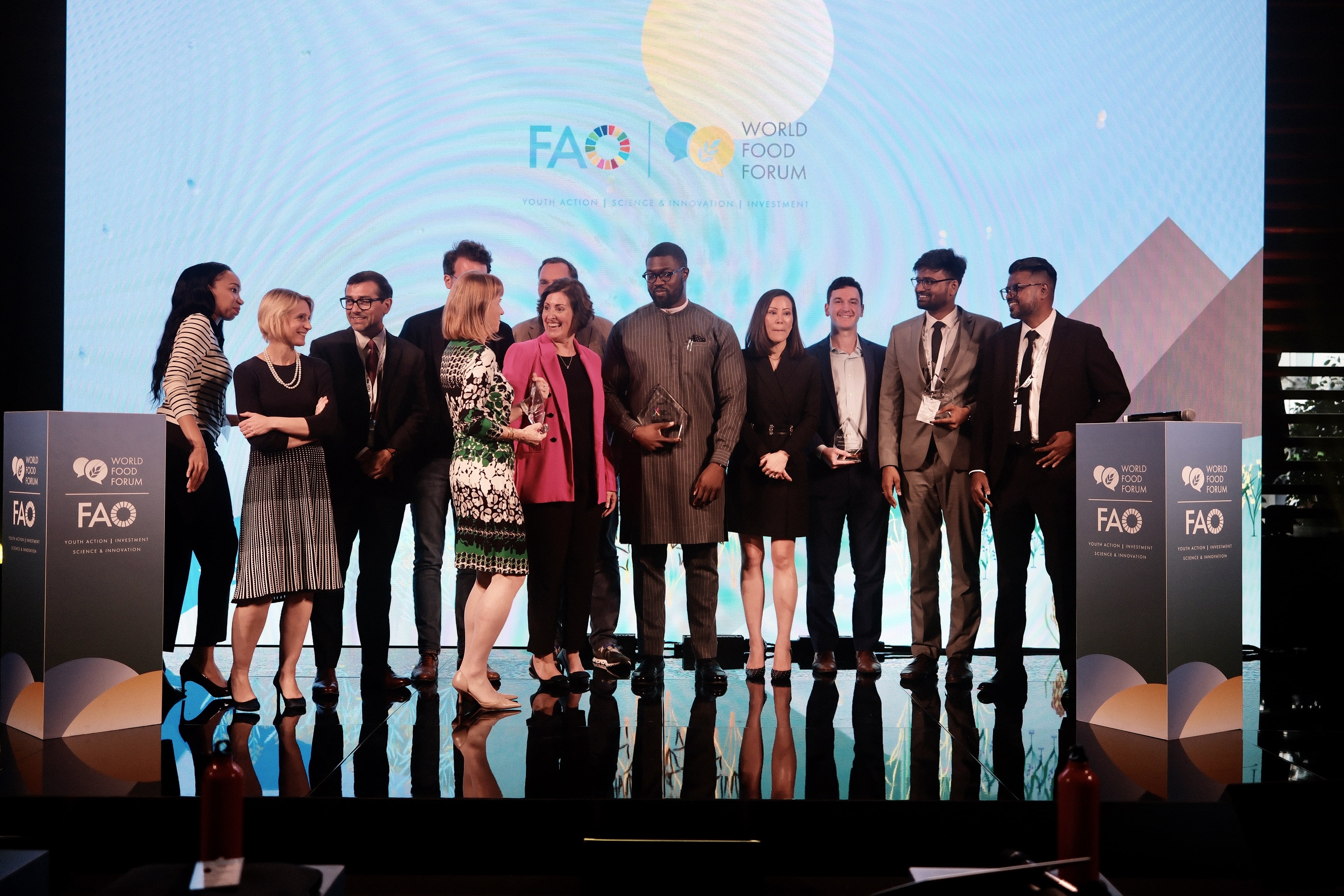The image captures a vibrant scene from an awards ceremony held during the World Food Forum. On the stage, an eclectic group of men and women, dressed in business attire, stand against a backdrop featuring the World Food Forum and FAO. The screen displays text promoting "Youth Action, Science and Innovation, and Investment." Among the diverse crowd are individuals of various races, including a black man, a white woman, and a Middle Eastern man, each proudly holding awards. The participants' smiles reflect their joy and the celebratory atmosphere of the event. Additionally, the stage is flanked by World Food Forum stand-up platforms and two red bottles of water can be seen offstage.